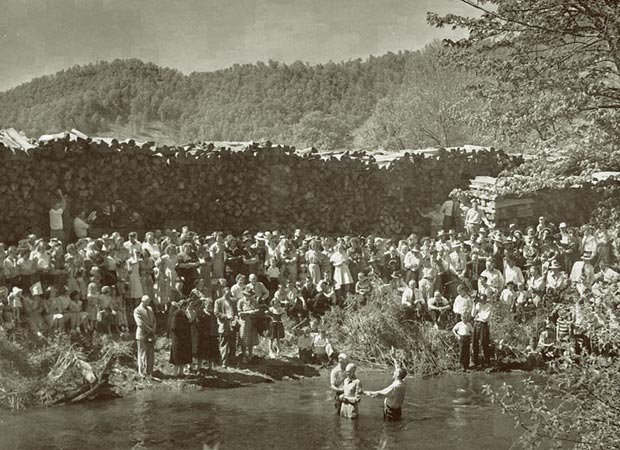This black and white photograph, taken in the Smoky Mountains, depicts a community gathering by a creek for a baptism ceremony. In the foreground, three clothed men stand in the water, with a preacher placing one hand on a man's shoulder and the other raised to the sky, surrounded by a congregation of about 200 people. The congregation lines the creek bank, standing behind a barrier of logs, suggesting the setting might be a logging camp. The background features dense trees, adding to the natural, serene atmosphere of the scene.